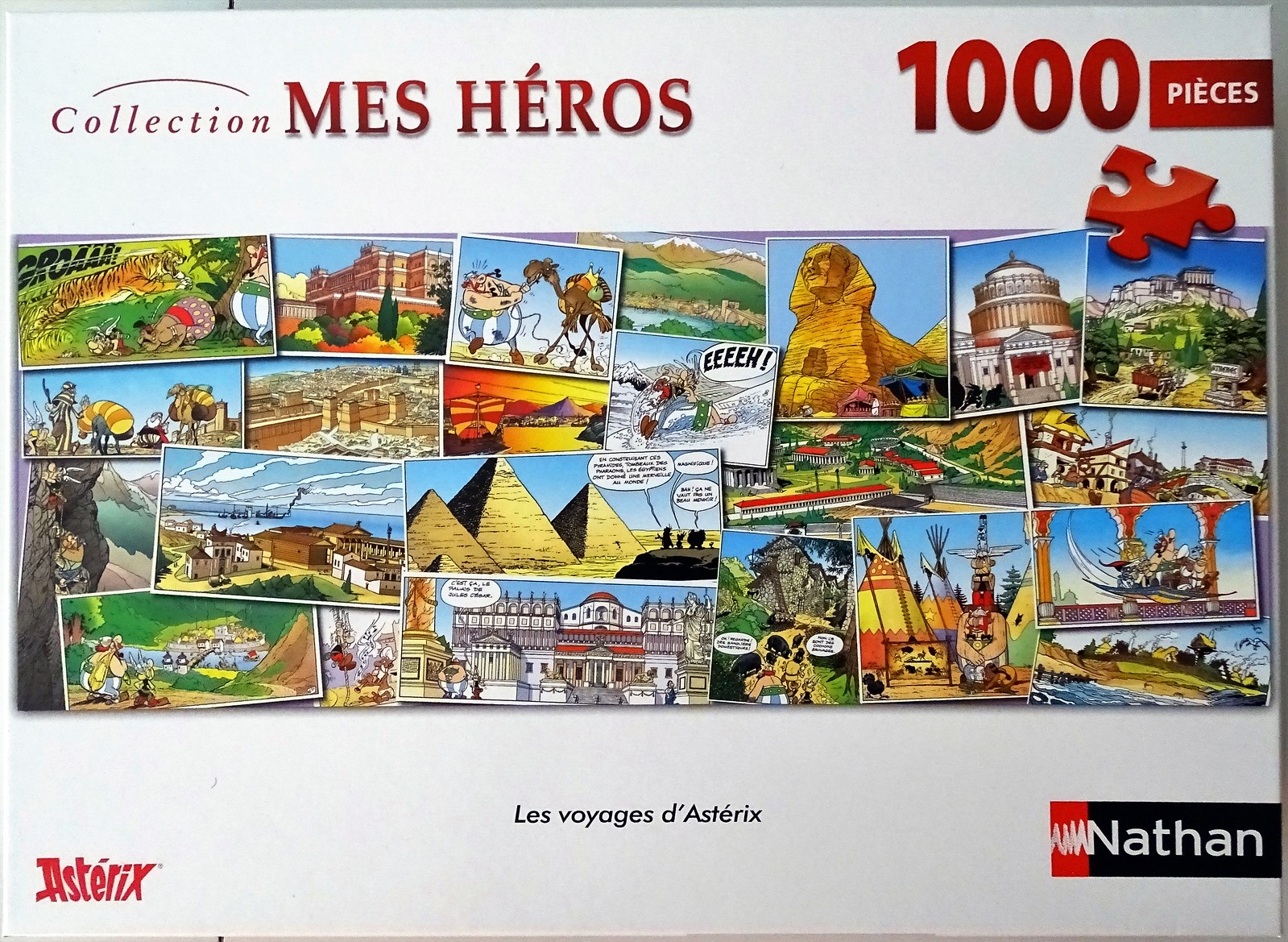This image depicts a 1,000-piece puzzle box from the "Collection Mess Heroes" series. The text indicating "1,000 pieces" is prominently displayed, with 'thousand' in black and 'pieces' in white on a black background. Below this, "Collection Mess Heroes" is written in black on a white background. The box features a vibrant collage of global landmarks and areas, including the tan Sphinx, the three Pyramids against a mostly blue sky, various tan buildings, and tigers with red and black stripes. Additional scenes include comic strips and an assortment of tourist destinations such as teepees. In the bottom left corner, "Asterix" is noted in red on a white background. Beneath the images, the text "Les Voyages d'Asterix" appears on a black and white background, along with the label "Nathan" in white on a black background, accompanied by a red and white symbol. This collection showcases puzzles depicting different parts of the world and famous locales, making for a colorful and detailed visual assortment.